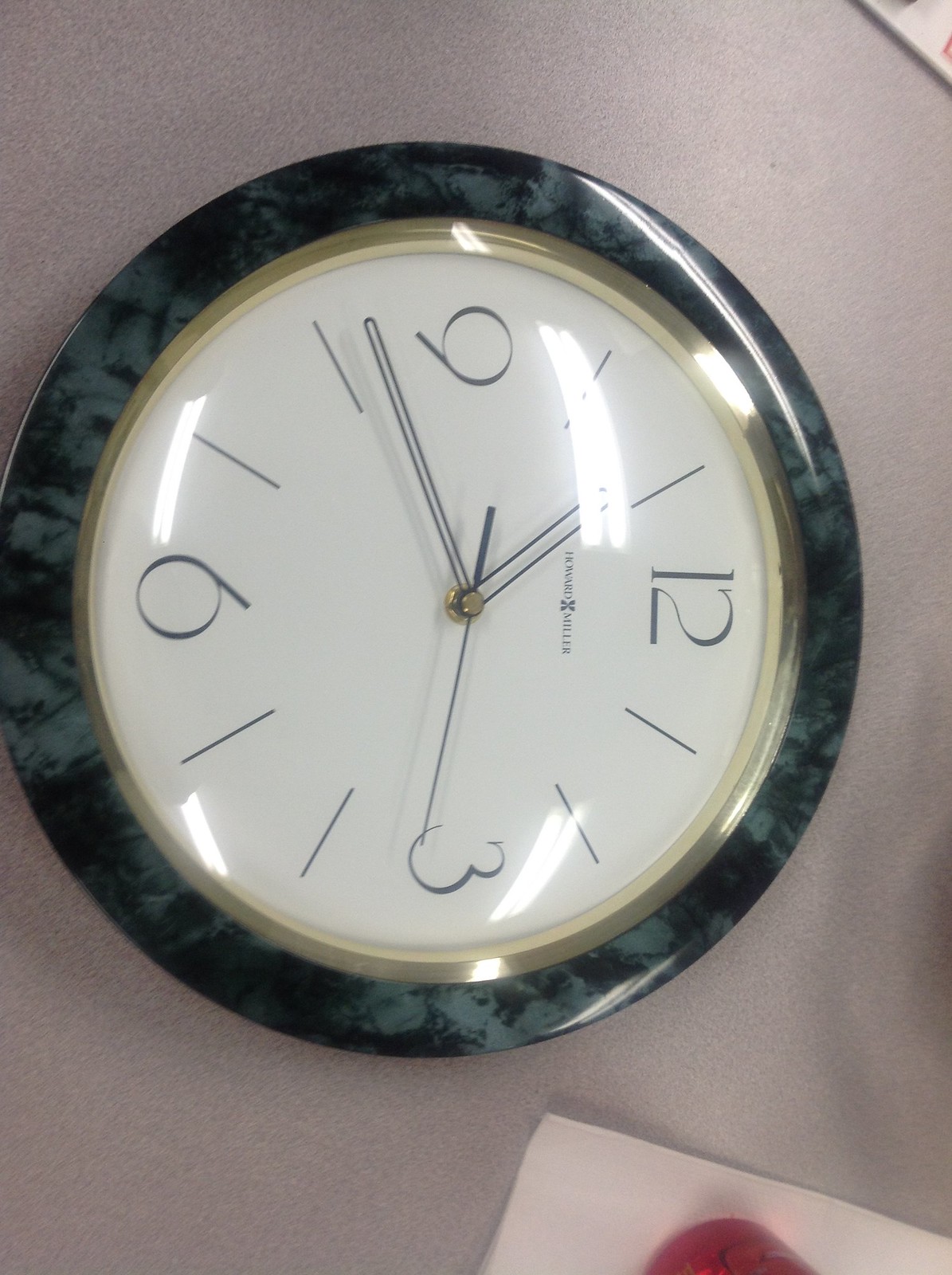In this rectangular image, the photograph is oriented sideways, showcasing a wall clock. The clock is turned such that the number 6 points west and the number 12 points east. The clock face is cream-colored with a green, marble-patterned border. The numerals 12, 3, 6, and 9 are displayed in black, while the remaining hours are represented by black tick marks. The timekeeping elements—a minute hand, an hour hand, and a second hand—are also black and centrally attached. The clock's face is encircled by a gold-colored rim, and a gold screw is visible at the center. This wall clock is mounted on a wall painted in a warm mocha color, complementing the elegant and classic design of the clock.